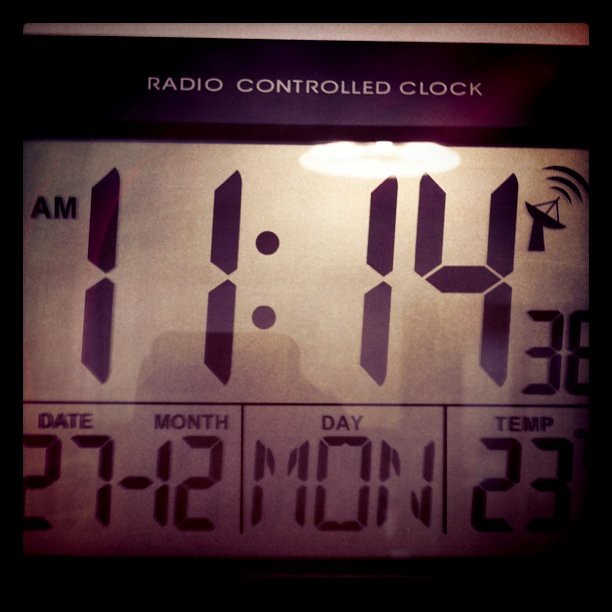This close-up photograph captures the display of a black, radio-controlled digital clock. Dominating the image is the large LCD readout showing the time as 11:14 AM. Above the time, small text identifies it as a radio-controlled clock, and an icon of a satellite with three radio wave symbols reinforces this feature. The date is displayed as December 27th, a Monday. The clock also indicates the temperature as 23 degrees. Reflections are noticeable on the glossy surface of the display, including the ceiling light fixture and the phone used to take the picture, although the photographer is not visible. The clock's plastic housing is mostly out of the frame, focusing the viewer solely on the detailed, informative display.